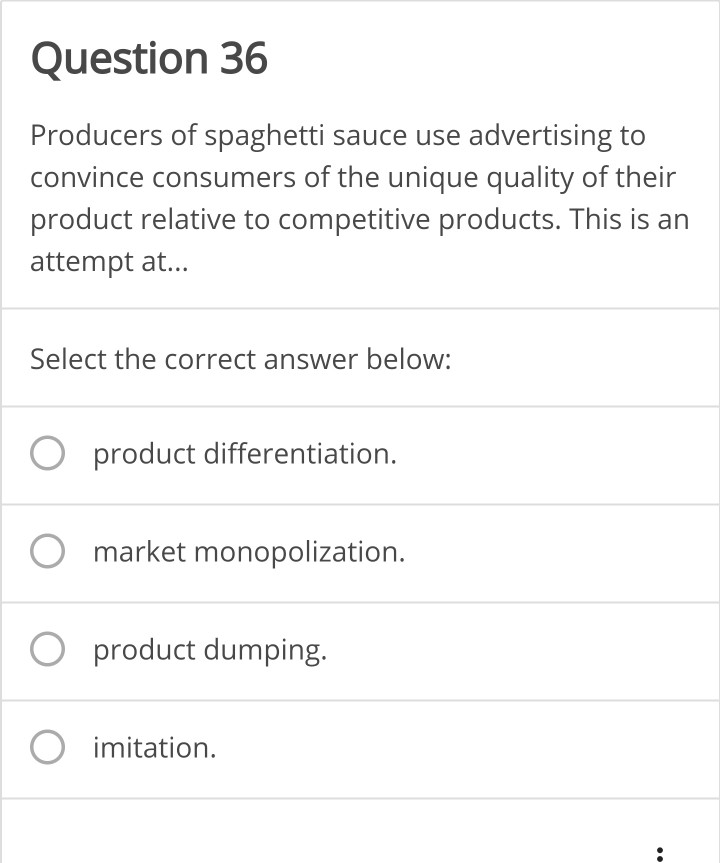This image is a screenshot of a digital test form displayed on a white background. The form is outlined by a subtle gray border and features gray-striped rows separating distinct sections. In the upper left-hand corner, the text "Question 36" is prominently bolded in black, with additional instructions underneath in gray font. The question reads: "Producers of spaghetti sauce use advertising to convince consumers of the unique quality of their product relative to competitive products. This is an attempt at."

Below the question, a prompt instructs the user to "Select the correct answer below," followed by four options, each accompanied by an empty white circle for selection. The options are:
1. Product differentiation
2. Market monopolization
3. Product dumping
4. Imitation

None of the options have been selected. At the bottom right-hand corner of the form, there are two small black dots, possibly indicating further options or a navigation element. This image captures the essence of a digital multiple-choice question, designed for the user to interact with by choosing the most fitting answer, which in this context is likely "product differentiation."